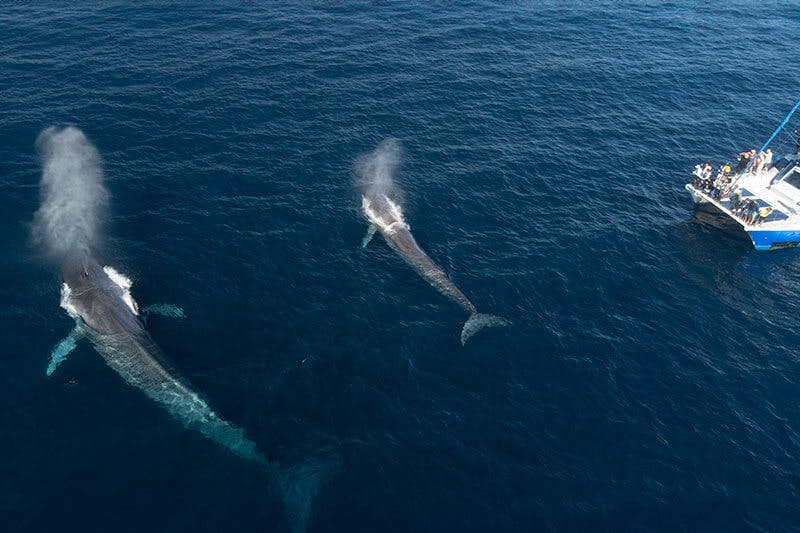An aerial photograph captures a serene, deep blue ocean scene with notable dark blue hues indicating the depth and light variations. In the left section of the image, two whales are surfacing and exhaling water through their blowholes, creating visible mist. The larger whale, likely a parent, dwarfs the smaller one nearby. The whale closer to the viewer showcases its front fins prominently, while the smaller whale’s tail fin is clearly visible. To the right side of the image, a white catamaran with a blue bottom and deck is filled with tourists, mostly gathered at the front, possibly taking photos or observing the majestic marine creatures. The boat appears sizeable but is overshadowed by the sheer size of the whales. The relatively calm waters add to the peaceful atmosphere of this open sea spectacle.